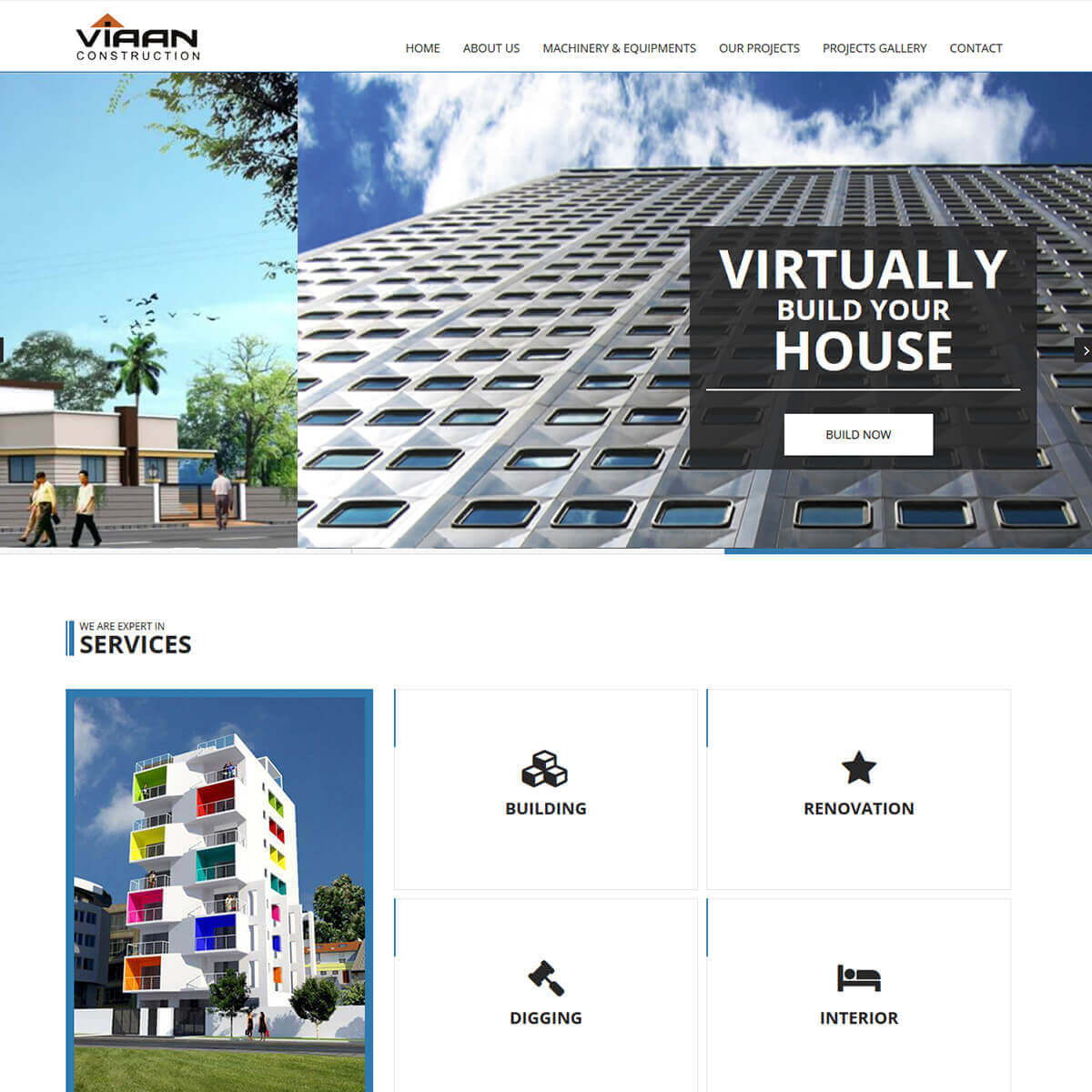This screenshot captures multiple aspects of Bayan Construction's projects and services. The main image showcases a massive building made primarily of metal, adorned with hundreds of small windows. Another image within the screenshot shows several people walking, with one individual preparing to enter a building. The scene is enhanced by a tall palm tree and birds flying across a clear sky. Cement steps lead up to the entrance, adding a touch of modern aesthetics. Additionally, there's an image of a vibrant high-rise building, possibly condos, featuring a white base accentuated with neon colors such as orange, blue, pink, yellow, and green. Text on the screen reads, "We are experts in services. Virtually build your house," along with a "Build Now" button. Service options listed include renovation, digging, interior design, and construction.